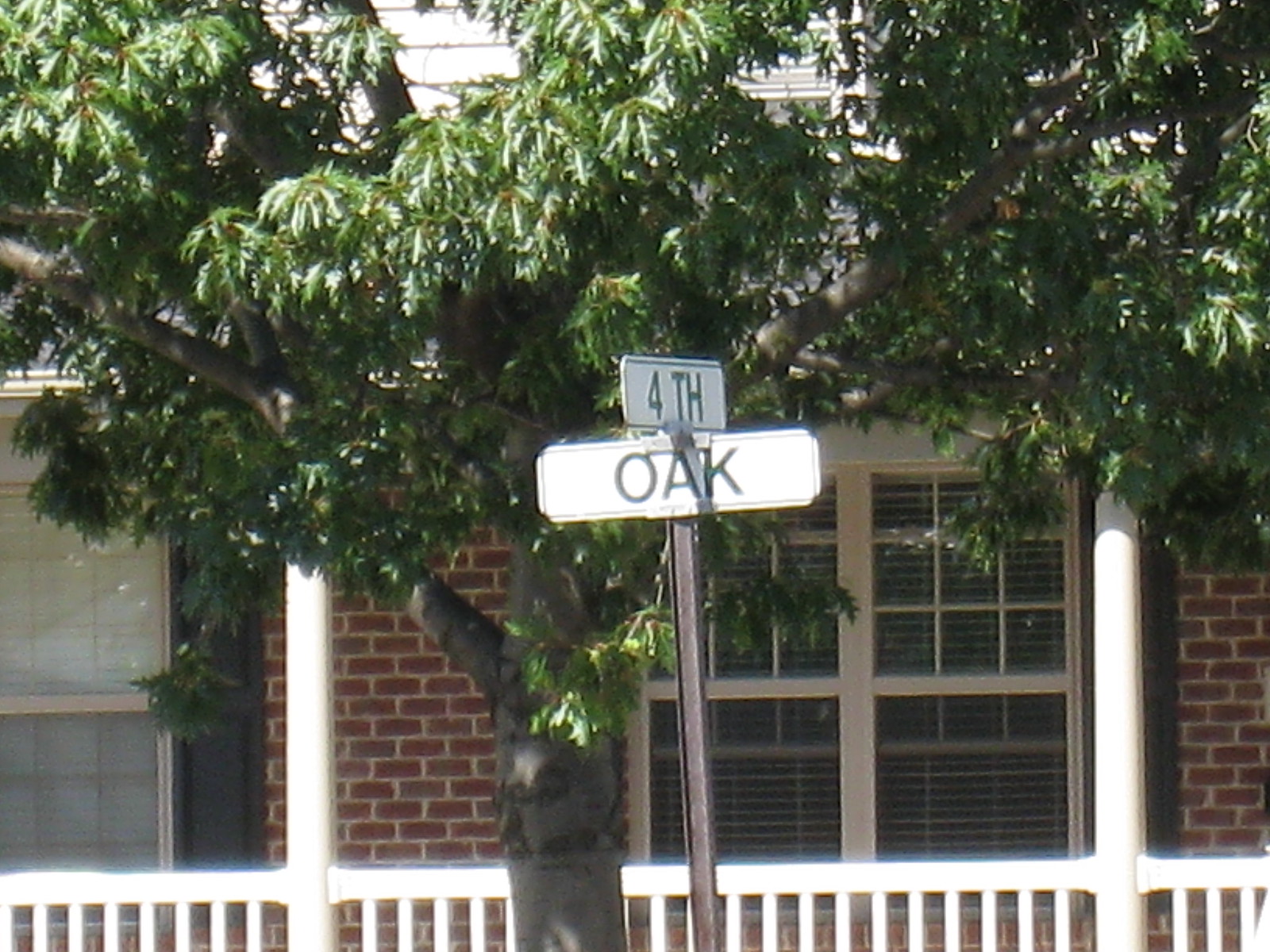The image showcases a street sign mounted on a pole, featuring two white rectangular plaques. The top plaque displays the word "Fourth" in dark green font, while the bottom one reads "Oak" in the same color. Behind the pole, a large tree with numerous branches and vibrant green leaves is visible. Situated further back is a brick house, which has a porch area accentuated with a railing. The house facade includes two windows; the right window has its blinds open, allowing a clear view, whereas the left window is adorned with curtains, keeping it closed.